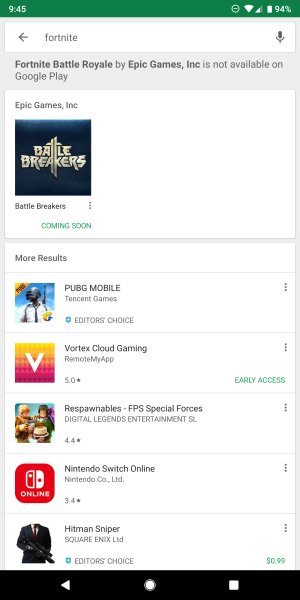This image is a screenshot of a mobile device taken at 9:45, as indicated by the clock on the top left. The top status bar features several icons: a WiFi icon, a cellular signal bar icon, a battery icon, and a battery percentage icon showing 94%.

In the main part of the screenshot, a search result for "Fortnite" is displayed. It states that "Fortnite Battle Royale by Epic Games Inc. is not available on Google Play."

Below this message, there are additional search results. The first listing is for "Epic Games Inc." followed by an icon labeled "Dale Breakers," which appears to be a game currently labeled as "Coming Soon."

Further down, more search results are shown, including:
- "Plank Mobile"
- "Vortex Cloud Gaming"
- "Respawnables FPS Special Forces"
- "Nintendo Switch Online"
- "Hitman Sniper"

At the bottom of the screen, a black navigation bar contains additional details. The "Editor's Choice" label is assigned to "Hitman Sniper." The following entry shows a 5.0-star rating described as "Easy Early Access," while "Respawnables" by Digital Legends Entertainment S.L. has a 4.4-star rating. "Nintendo Co. Ltd" is listed with a 3.4-star rating.